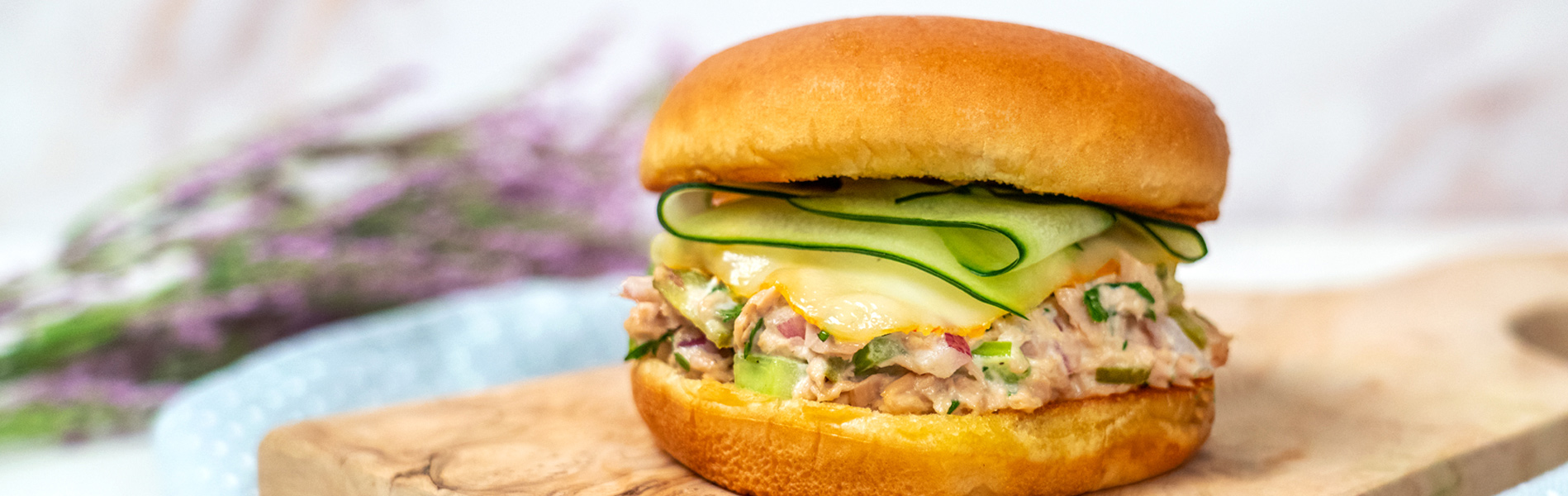This is a detailed close-up photograph of what appears to be a vegetable sandwich, presented on a golden yellow potato bun that rests on a wooden cutting board. The sandwich sits on what looks like a glass table, with a background that is intentionally out of focus, revealing glimpses of purple flowers and possibly some green foliage.

The top layer of the sandwich showcases very finely sliced, curled cucumber, contributing a fresh and crisp element. Below the cucumber resides a layer of white cheese, which appears to be either slightly melted or simply nestled into the creamy salad mixture beneath it. This salad mixture, which forms the core of the sandwich, looks somewhat gloppy and creamy, suggesting that it could be a chicken salad, tuna salad, or possibly even a salmon salad, denoted by its pinkish hue. Inside this mixture are identifiable elements such as green bits, possibly celery, and purple onions, giving the sandwich a varied texture and flavor profile. There's speculation that the salad mix might contain potato as well, adding to its heft.

The sandwich’s bottom bun completes the stack, contributing to what some might consider an overall unappealing presentation. The sandwich appears a bit messy, with the salad mixture generously spread and perhaps seeping out from the sides, giving it a sloppy appearance. Despite the detailed layers and elements, the sandwich, with its vibrant mix of greens and the crispy potato bun, presents an intriguing if somewhat controversial visual appeal, especially given its setting amidst the colorful, blurred background.